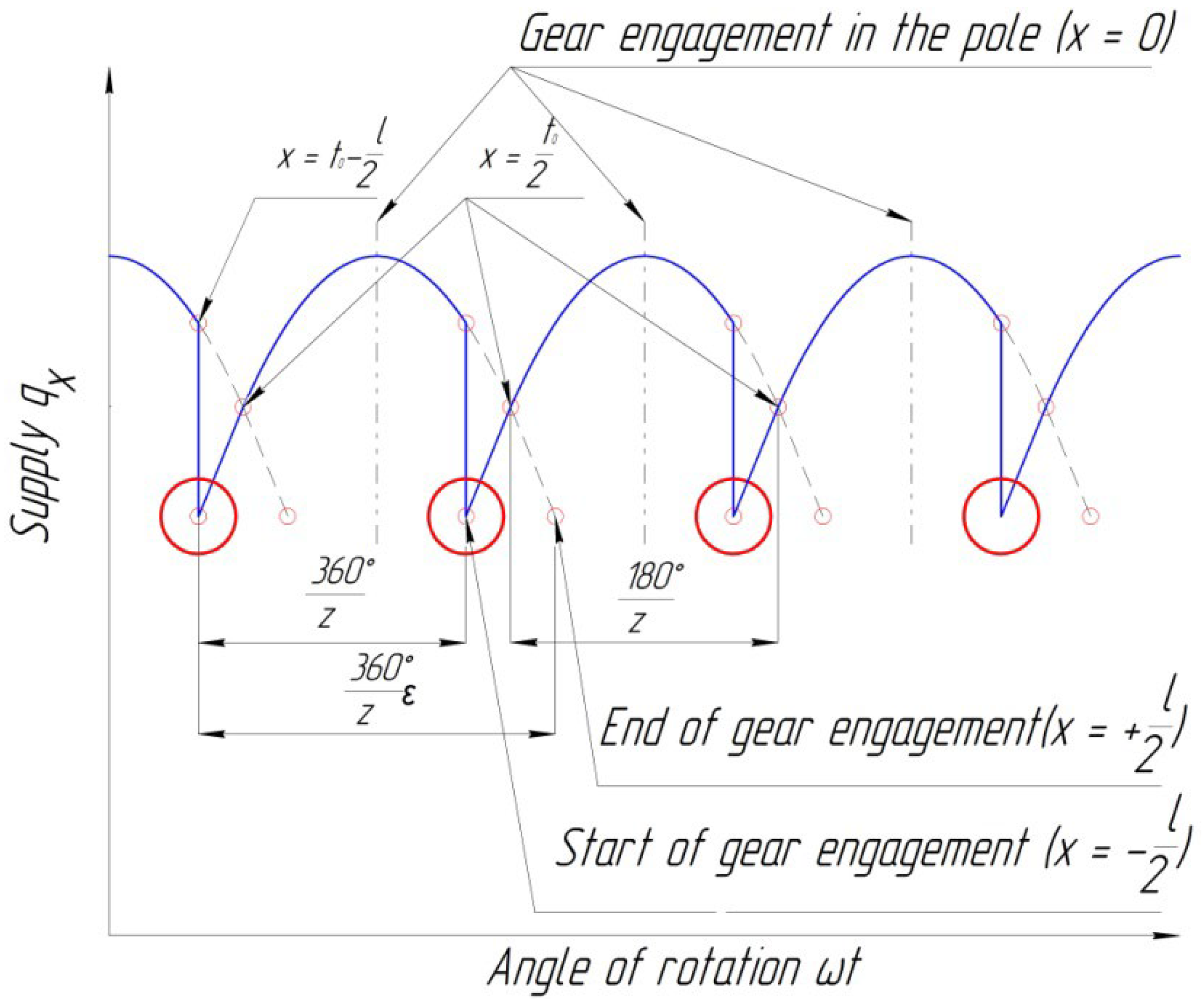The image depicts a detailed mathematical graph illustrating gear engagement in a pole. The primary colors featured are red, blue, and black. At the center of the graph, various equations and labels are prominently displayed. The x-axis is titled "Angle of Rotation (WT)", while the y-axis is labeled "Supply (QX)". Key annotations include "End of Gear Engagement (x = +1/2)" and "Start of Gear Engagement (x = 1/2)". Other notable equations present are "X = T0 - 1/T", "X = T0/2", "360 degrees/Z", and "180 degrees/Z". The graph features blue curves with red circles highlighting specific points along the valleys, indicating critical points of gear engagement and disengagement. The overall style and setting reflect a complex mathematical problem or question.